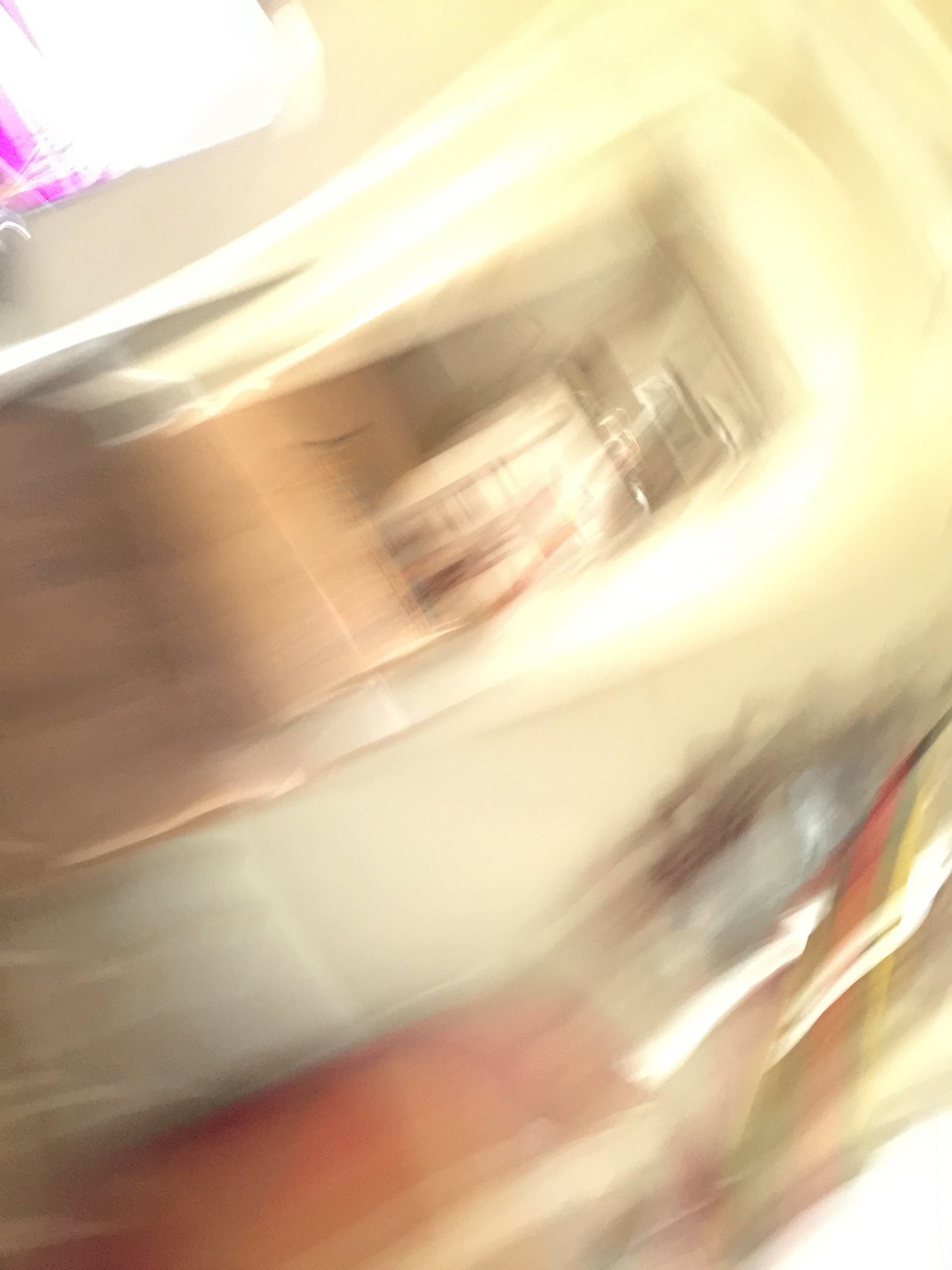This incredibly blurry image appears to be taken inside a home, capturing various elements in a state of motion. In the far upper left, a bright area suggests natural light, possibly from a window, next to which there's a visible purple triangle adjoining a white rectangle. Moving right, a light brown strip transitions into a yellowish-brown band. Across the center are white horizontal strips, beneath which a brown cylindrical object with protruding white lines connects to a dark patch. Central to the photo is an opening that might be a door frame, showcasing a silver background. The bottom half, especially the right side, contains a mottled array of colors—blacks, grays, bright whites, and a reddish-gray hue—suggesting a high-speed movement. A bluish-gray fragment and a transitioning brown-to-blue element hint at diverse textures and materials. Some details resembling walls, picture frames, and a lampshade give context to the indoor setting, despite the overwhelming blur.